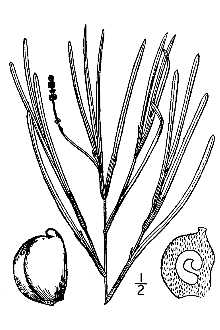This detailed black and white pencil or black ink and pen drawing showcases a small, stocky plant with an intricate central stem from which approximately a dozen slender branches extend. These branches resemble mini stems rather than traditional leaves. Positioned at the base of the plant, the drawing includes two detailed depictions of a fruit, nut, or seed that likely grows on this plant. On the bottom left, there is a whole representation of this item, while on the bottom right, a cross-sectional view reveals the interior structure with visible seeds and a central core. Between these two depictions, centrally aligned at the base, is the fraction “1/2”, indicating the cross-sectional nature of the right-side illustration. The background is white, emphasizing the careful and delicate lines of the drawing.